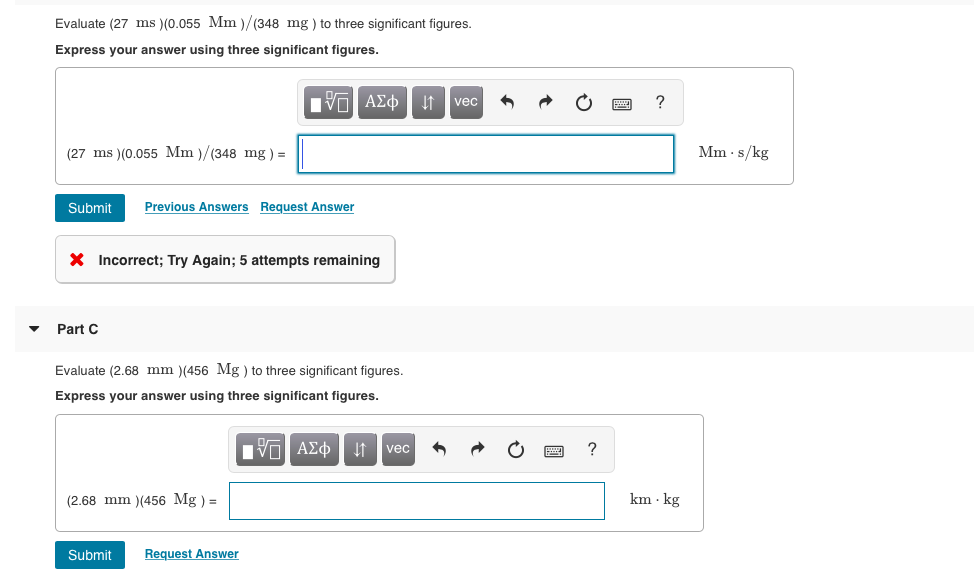The image displays a section of an educational or calculation application. The screen presents a problem requiring the evaluation of a mathematical expression and entry of the result to three significant figures. 

### Details of the Image:

- **Header Section**:
  - Likely shows part B of a problem, with the top of the screen partially visible.
  - Contains an equation: \( 27 \, \text{MS} \times 0.055 \, \text{mm} \div 348 \, \text{mgs} = \), with a box for inputting the answer.

- **Middle Section**:
  - Underneath the equation, there is a teal button labeled "Submit."
  - Additional options in teal include "Previous Answers" and "Request Answer," both underlined.
  - A gray box with text stating "Incorrect. Try again. Five attempts remaining" is present, accompanied by a red 'X' icon. 

- **Lower Section (Part C)**:
  - Clearly marked as "Part C."
  - Instructions are given to evaluate \( 2.68 \, \text{mm} \times 0.456 \, \text{mgs} \) to three significant figures.
  - The text instructs to express the answer using three significant figures.
  - Displays the equation: \( 2.68 \, \text{mm} \times 0.456 \, \text{mgs} = \), with a box outlined in blue for the input.
  - Two blue buttons labeled "Submit" and "Request Answer" are shown next to it.

Overall, the application guides the user through the process of solving and submitting answers, with feedback provided on their attempts and clear instructions for the required precision and format.